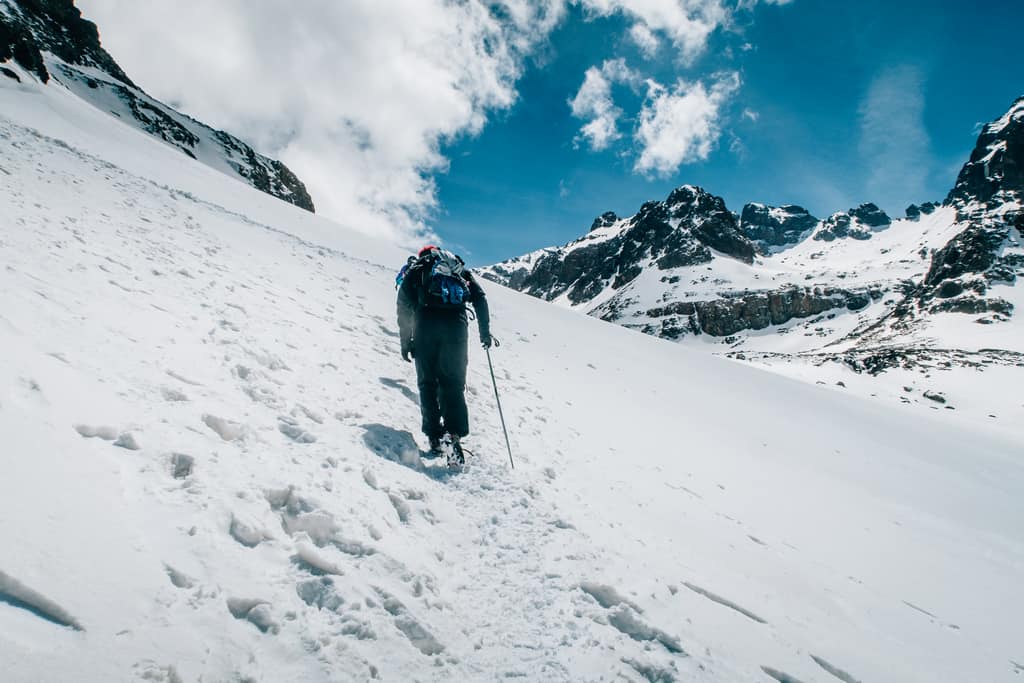In this image, we see a photograph of a man hiking up a snow-covered mountain slope. The scene captures the rugged and icy terrain of the mountain range, with the elevation sloping steeply down on the right and sharply upward on the left, creating a dramatic contrast. The densely packed snow blankets the entire landscape, with clearly visible footprints dug into the snow. The hiker, dressed in a thick winter jacket, black snow pants, and boots equipped with ice grips, trudges through the challenging terrain aided by a metal walking pole. To the right, the mountain range extends into the distance, featuring dark gray, jagged rocky cliffs topped with snow. The sky above is an aqua blue on the right side, gradually giving way to thick white clouds on the left, creating a striking and picturesque backdrop for the arduous climb.